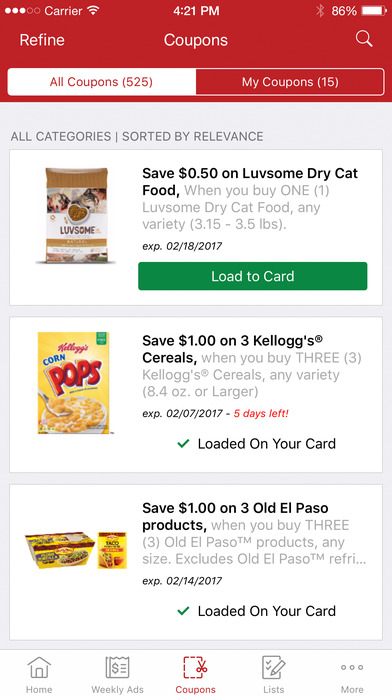This image showcases a coupon app interface. At the top, there is a red box containing the white text "Refine" and "Coupons". Within this red box, a white sub-box displays "All Coupons (525)", indicating there are 525 available coupons, and next to it, "My Coupons (15)" suggests 15 saved coupons. Below, the app allows navigation through "All Categories" and is sorted by "Relevance".

The first visible coupon offers savings of 50 cents on "Love Some Dry Cat Food" when purchasing any 3.5-pound variety. A green "Load-to-Card" button is available beneath this offer.

The second coupon provides a $1 discount on three Kellogg's cereals of any variety, 8.4 ounces or larger. This coupon expires on February 7, 2017, denoting that the image was captured in 2017, and it shows that the coupon is already "Loaded on your card" with a green checkmark indicating its status.

Another coupon offers $1 off three Old El Paso products, excluding some specific varieties. This coupon also indicates it has been "Loaded on your card" and has an expiration date of February 14, 2017. Some text is partially cut off, but essential details remain readable.